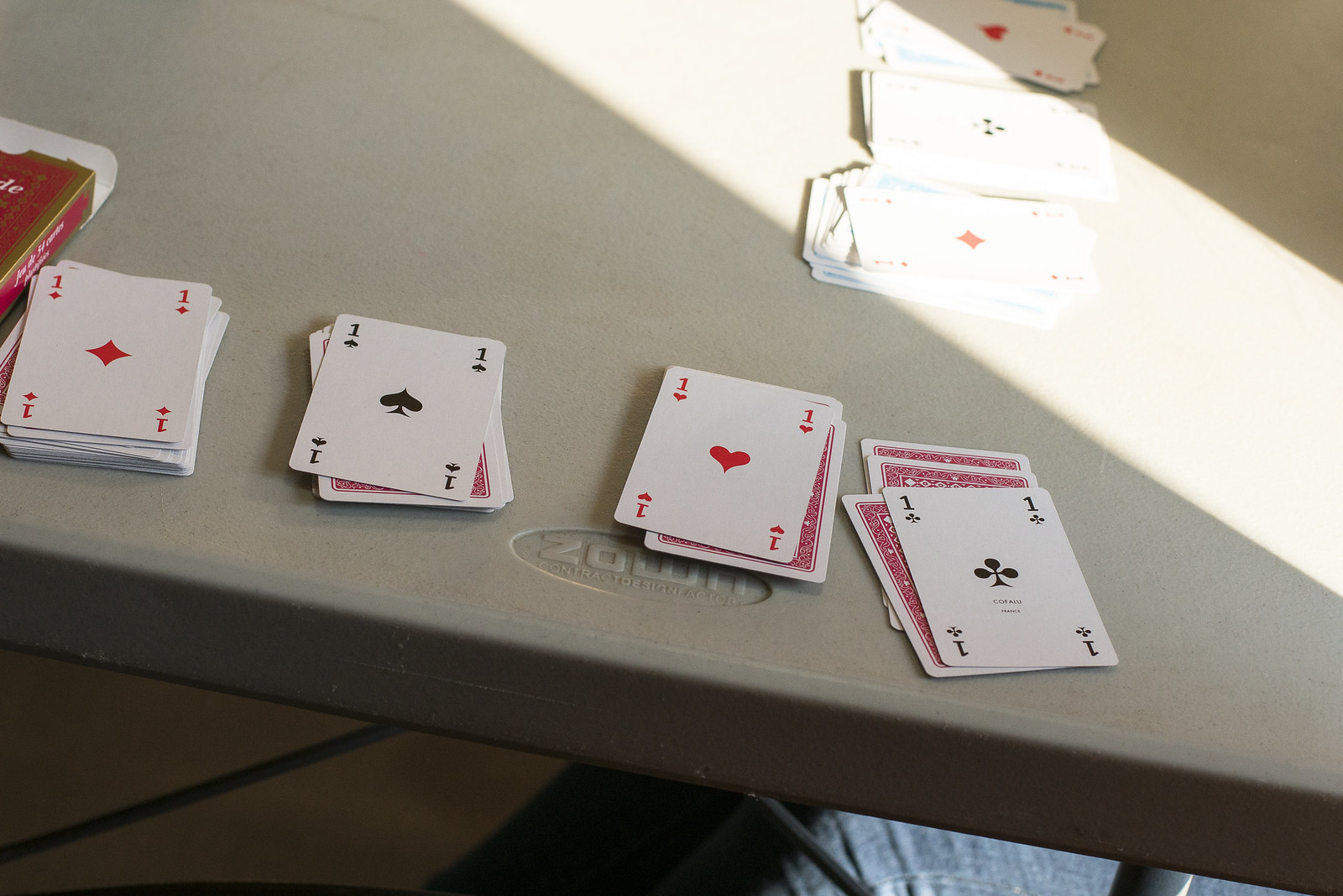In the close-up image, two decks of cards are split into neat yet slightly scattered piles on the edge of a foldable plastic table. The focal point is the four visible aces crowning each of the four piles of cards on the left side: from left to right, the ace of diamonds, the ace of spades, the ace of hearts, and the ace of clubs. Parallel to these piles, another deck is also split into four stacks at a right angle, with three aces visible: the ace of diamonds, the ace of clubs, and the ace of hearts. The fourth pile's ace is out of frame. Only the edge and a bit of the tabletop's legs are visible in this close-up shot, emphasizing the carefully arranged arrangement of the cards.